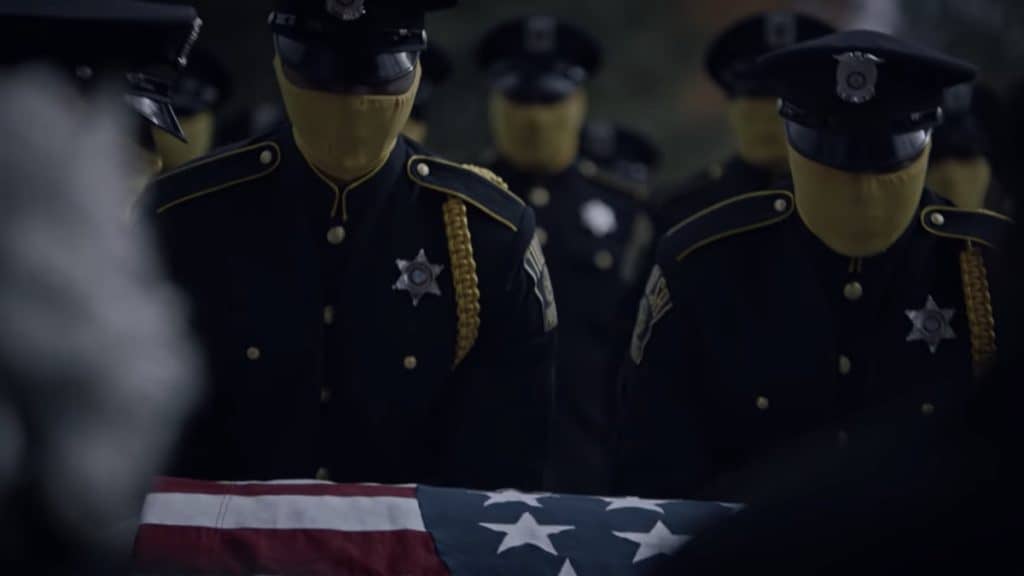The image depicts a solemn scene of police officers or servicemen, possibly attending a funeral ceremony for a fallen comrade. At the forefront, a group of officers is seen carrying a casket draped with an American flag, displaying the blue field with white stars and the red and white stripes. The officers are dressed in dark blue uniforms adorned with gold epaulets, ropes around their shoulders, and six-pointed silver sheriff stars on their left chests. Their uniforms also feature gold pinstriping on the shoulders and circular gold buttons down the front. The officers wear blue hats with silver badges and black brims. Curiously, all the officers' faces are obscured by yellow face coverings, rendering them almost faceless, with only an eerie emptiness where their expressions should be. At the front, some officers lean slightly downward, while others in the background stand straight in a precise formation. The image has a computer-altered appearance, further emphasizing the featureless faces of the officers.